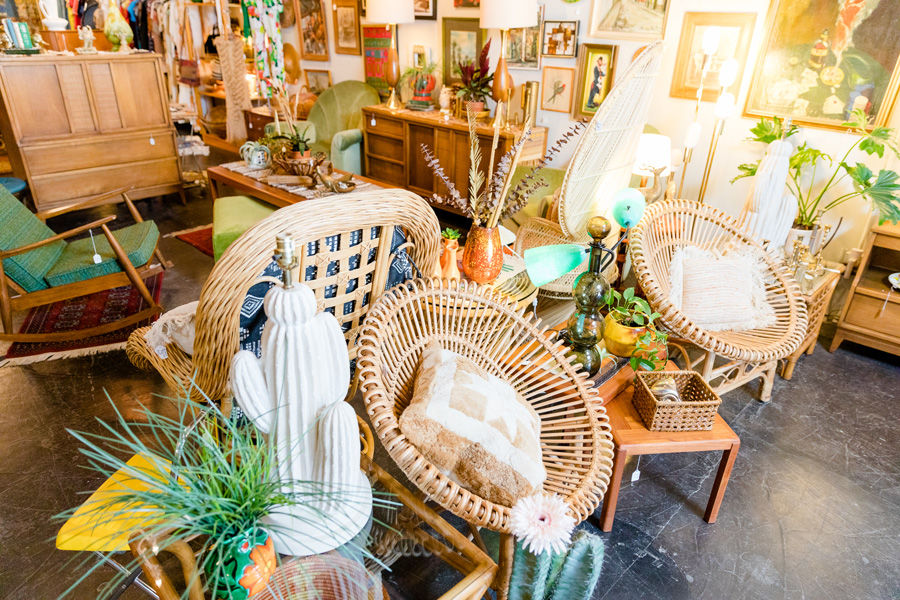The image depicts the interior of an eclectic home goods store, vividly filled with a diverse array of furniture and decorative items. In the foreground, two unique wicker chairs, each with plush tan and white pillows, are positioned diagonally to the viewer. These chairs flank side tables topped with distinct marble-like cacti lamps. The store’s aesthetic features a harmonious mix of natural materials and colors, such as wicker, wood, greens, browns, and yellows, evoking a cozy, vintage vibe reminiscent of a grandparent’s house.

Throughout the store, additional seating options include matching wicker chairs and several rocking chairs with green cushions, contributing to the inviting atmosphere. Among the furniture, there are wooden dressers and bureaus, one with two rows of drawers and an intriguing thick rectangular top, suggesting functionality. The store also displays scattered rugs, including a red mosaic rug with white fringes.

The walls are adorned with an assortment of paintings in various styles and colors, ranging from reds and blues to pinks and yellows. These artworks include both faded pieces and vibrant abstracts. A section of the store hints at a clothing area, visible in the left-hand corner, adding to the space's charmingly cluttered ambiance.

Surrounded by various plants, including striking cacti or ceramic-like cactus structures, the store bursts with life. The floor appears to be a cracked, blue-black cement, adding a rustic touch to the overall setting. The detailed and colorful environment makes this store a treasure trove of home goods and decorative treasures.